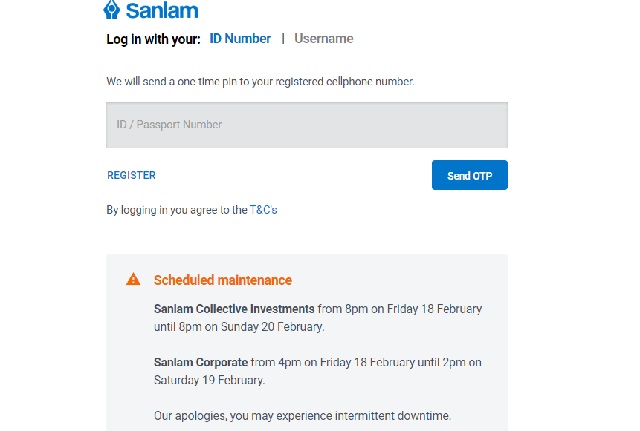The image features a white background with a blue header at the top. Within the blue header, there is a blue logo accompanied by the text "Send LAMB." Below the header, the text prompts users to "log in with your ID number or username," with the phrase "ID number" highlighted in blue for emphasis. Further down, an instruction reads, "We will send a one-time PIN to your registered cell phone number."

A light gray text box is displayed beneath this instruction, featuring the placeholder text "ID/passport number." Directly below this text box is a blue button labeled "Send OTP," and to its left, a link that says "Register." The bottom part of the image includes a note stating, "By logging in you agree to the TUCs."

Towards the lower section, there is a gray box with a red triangle containing an exclamation mark, indicating an alert. This box warns of "scheduled maintenance" in red text and further clarifies in black text that Send LAMB collective investments will be undergoing maintenance from 8 p.m. on Friday, February 18th, until 8 p.m. on Sunday, February 20th.